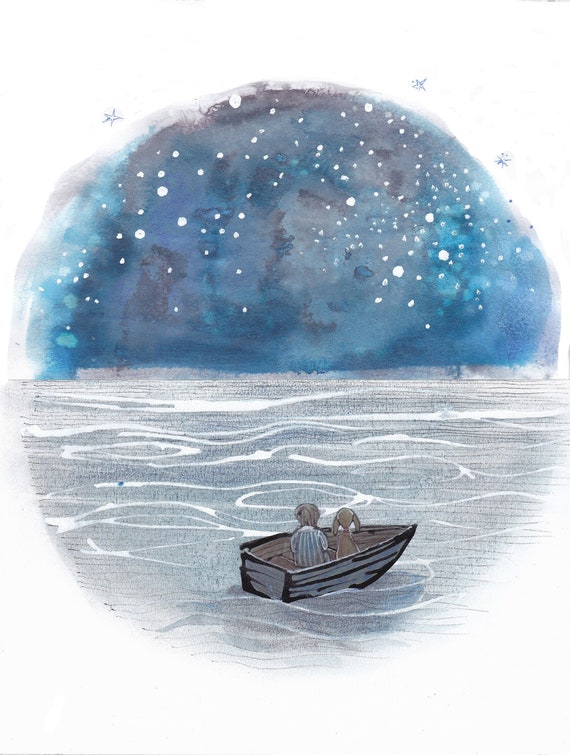This watercolor-style illustration is centered on a blank white canvas. The artwork is enclosed within a circular frame that fades into the surrounding white background. The top half of the circle depicts a dark and mottled blue night sky dotted with numerous white specks, resembling stars. Just outside the circle, three blue-outlined stars are also visible.

The bottom half of the circle portrays grayish-blue water adorned with swirling white outlines. Floating on this water is a small, pointed wooden boat oriented to the right. Inside the boat, a young boy with short brown hair, clad in a blue and white vertically-striped pajama shirt, sits on the left side, while a brown dog with long ears and a red collar sits to his right. Both the boy and the dog are seen from behind, gazing out over the water into the expansive sky, adding a sense of wonder and tranquility to the scene.